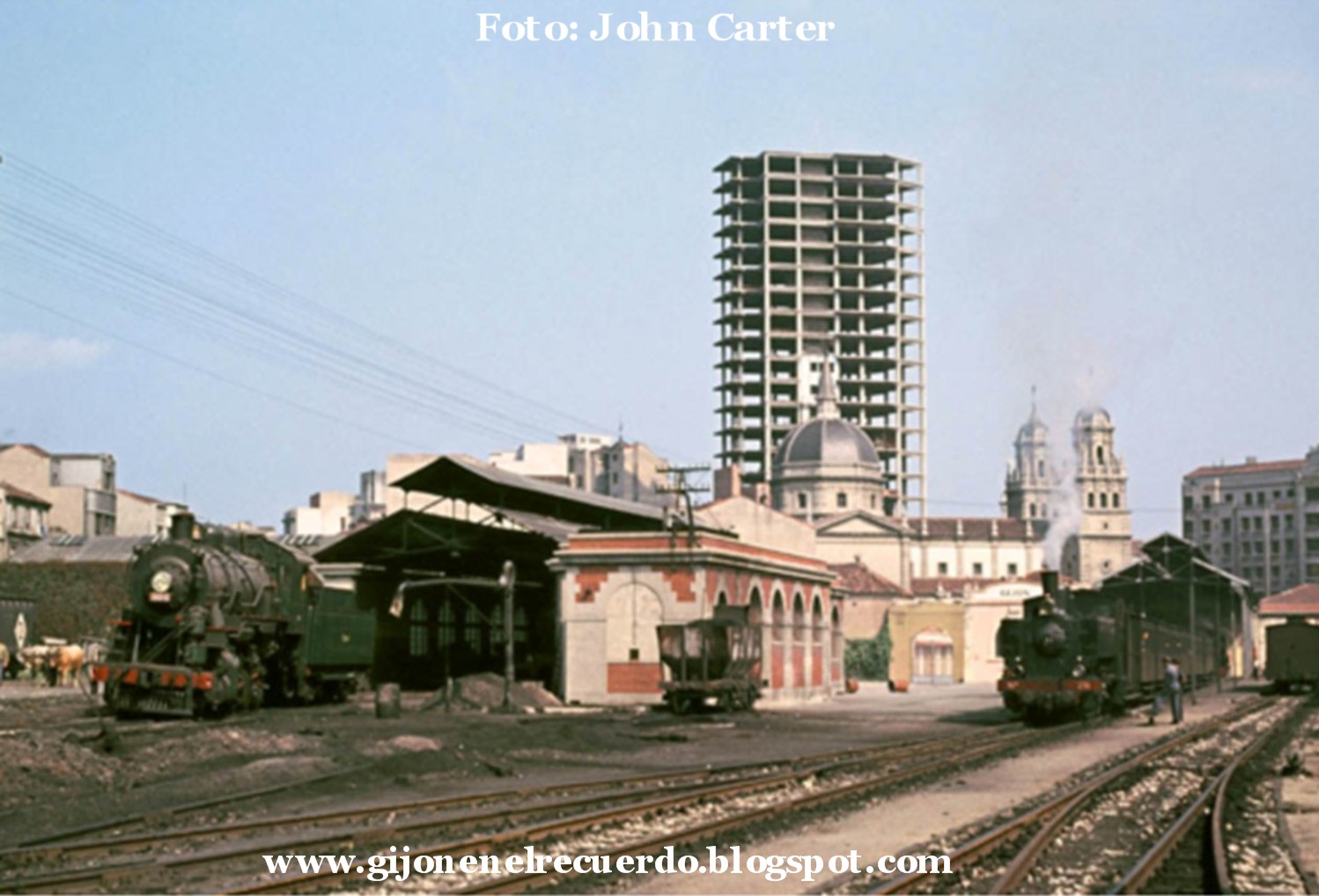In this evocative photograph titled “Foto: John Carter” (top) and labeled at the bottom with www.gijonercuerdo.blogspot.com, we peer into an industrial railyard scene, seemingly set in the 1970s somewhere in Eastern Europe. The foreground prominently showcases two vintage steam trains; the one on the left is green while the right one is red, resting majestically on the tracks. The front of the green train appears to be covered in ivy, adding a touch of nature to the industrial setting. 

To the left, the scene is anchored by old-fashioned brick buildings and industrial warehouse structures, while the right side is dominated by a mix of architectural elements. Among them, a building with a distinctive dome ceiling topped by two smaller dome towers rises, possibly a church. Adjacent to this, a tall, eight-story apartment building with an Eastern European or Turkish style ascends into the clear, blue sky, intersected intermittently by electrical wires. In the background, the skeletal framework of a skyscraper looms, partially built with visible concrete and steel, hinting at development and modernization amidst the historical backdrop. This vivid contrast between old and new, nature and industry, transports viewers into a nostalgic tableau of urban life during a transformative era.